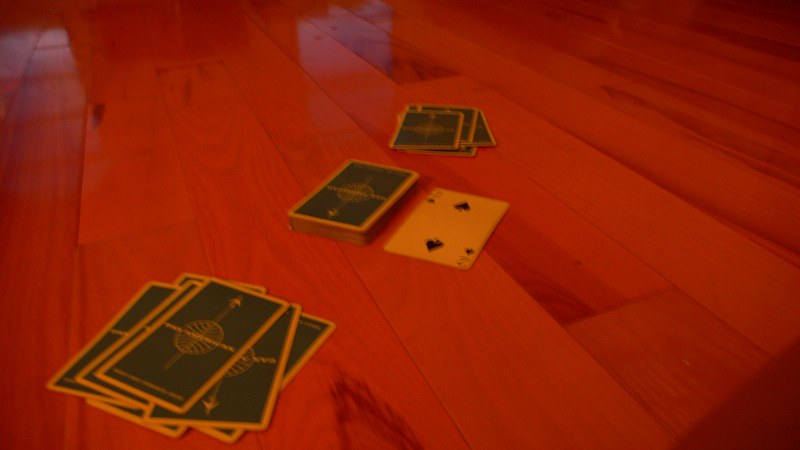In this image, we observe a dimly-lit card game in progress, bathed in a warm yellow glow that casts a cozy yet blurry atmosphere over the scene. The playing surface is a wooden table characterized by wide, evenly spaced, lacquered slats, though it could potentially be a wooden floor, given its extensive appearance. Two players are engaged in the game, with a face-down stack of cards placed centrally between them. On top of this stack rests the two of spades and another indistinguishable card. The player closest to the camera has a disorganized face-down pile of approximately 7 or 8 cards. Across from them, the opposing player holds a similarly untidy stack of about 5 face-down cards. The overall setting exudes a sense of intimacy and casual engagement, with the subdued lighting adding to the scene's warm, inviting ambiance.